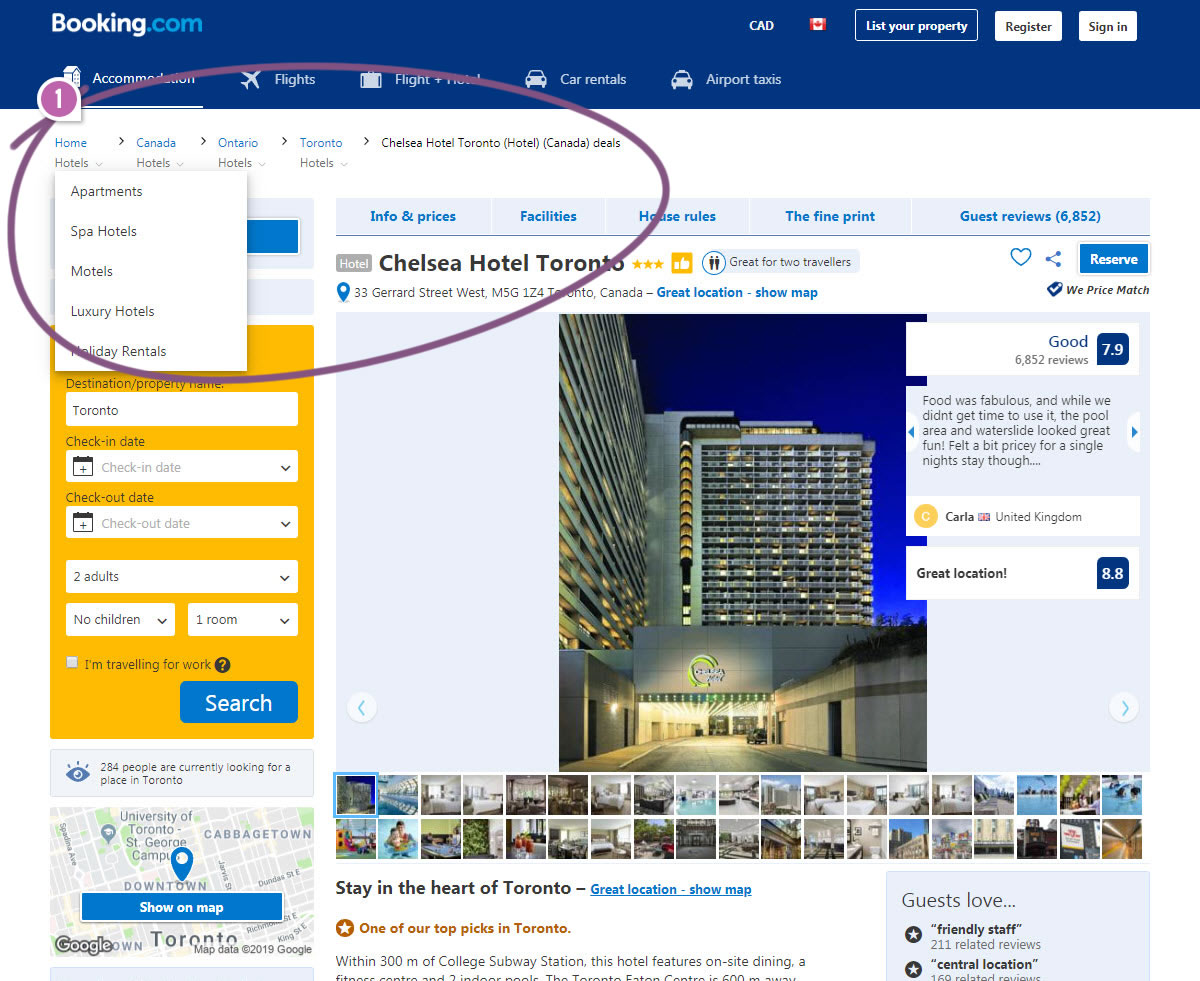The image features a detailed booking interface for Chelsea Hotel Toronto on the Booking.com website. 

At the top of the screen, there's a long blue rectangle that prominently displays the white text "Booking" followed by the light blue ".com". Beside this, "CAD" is written, indicating Canadian currency. Towards the right, there's a red and white symbol that is not clearly identifiable, followed by a white-outlined rectangle containing the text "List Your Property". Another white rectangle beneath this reads "Registration", and next to it is "Sign In".

A large purple circle, outlined in white, is positioned prominently on the screen, inscribed with "One" inside. To the right of this circle, there is a breadcrumb navigation path showing: Home (in blue) > Canada > Ontario > Toronto > Chelsea Hotel Toronto > Hotel Canada Deals (in black).

Below this, a white rectangle lists the different property types - "Apartments, Spa Hotels, Motels, Luxury Hotels" and "Holiday Rentals", though partly obscured. A yellow rectangle, partly overlapped by a white rectangle, contains unreadable small text. Next, there's a white rectangle labeled "Toronto" and another with a small calendar symbol that says "Check the Date". Two more white rectangles respectively read "Check-In Date" and "Check-Out Date".

Underneath these, there's a white rectangle indicating "2 Adults", followed by another saying "No Children" and "1 Room". Additional illegible text is present in smaller fonts. A blue rectangle containing "Search" is highlighted at the bottom.

Further down, light green or blue text that's too small to read is accompanied by a map-like visual, followed by a blue rectangle that states "Show on Map". Moving right, there's a light blue rectangle with indistinct text. Below that, the background shifts to white and black, displaying "Chelsea Hotel Toronto" in bold. Adjacent to this are a grey rectangle with the text "Hotel" and several yellow stars, a yellow box with a white thumbs-up icon, a circle with two people inside, and additional text. Also present are a blue-outlined heart, a share button, and a blue rectangle that says "Reserve".

Below these elements, an address is denoted with a map pin icon, and text "Great Location" and "Show Map" highlighted in blue. An image of the Chelsea Hotel Toronto is displayed, followed by a series of smaller pictures. Accompanying the photo montage, in bold font, is "Stay in the Heart of Toronto. Great Location. Show Map.", with "Great Location" and "Show Map" emphasized in blue.

In brown, a circle with a white star inside announces, "One of Our Top Picks in Toronto". Underneath, there's additional black text, followed by a blue rectangle titled "Guests Love". Two blue circles with stars and words denote positive attributes: "Friendly Staff" and "Central Location".